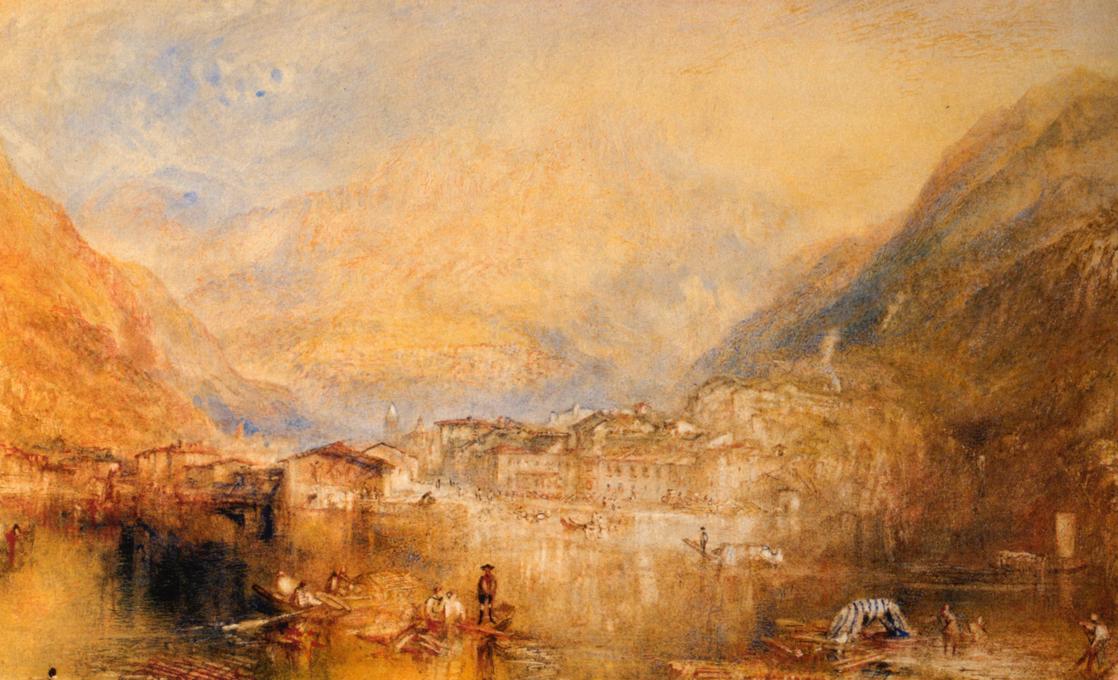This detailed watercolor painting, titled "Brunnen from the Lake of Lucerne" by Joseph Mallard William Turner, completed in 1845, vividly portrays a serene lakeside village nestled within a mountainous valley. The predominant colors are muted browns, rust oranges, and deep goldenrod yellows, with touches of cyan blue peeking through the sky and the reflective lake surface.

In the foreground, a tranquil scene unfolds at the water's edge, where several figures are engaged in various activities. Some are aboard slender, gondola-like boats, possibly barges, equipped with oars. Notably, a man wearing a black hat and black pants stands prominently in one of the boats, facing the viewer. Other individuals on the shore are busy with their daily work, near a small striped shelter resembling a tent.

The village, situated at the far edge of the lake, features two-story buildings that climb slightly up the mountainside, blending seamlessly into the muted landscape. The background is dominated by tall, indistinct mountains, their outlines blurring into the soft, overcast sky, enhancing the painting's overall subdued and harmonious aesthetics.